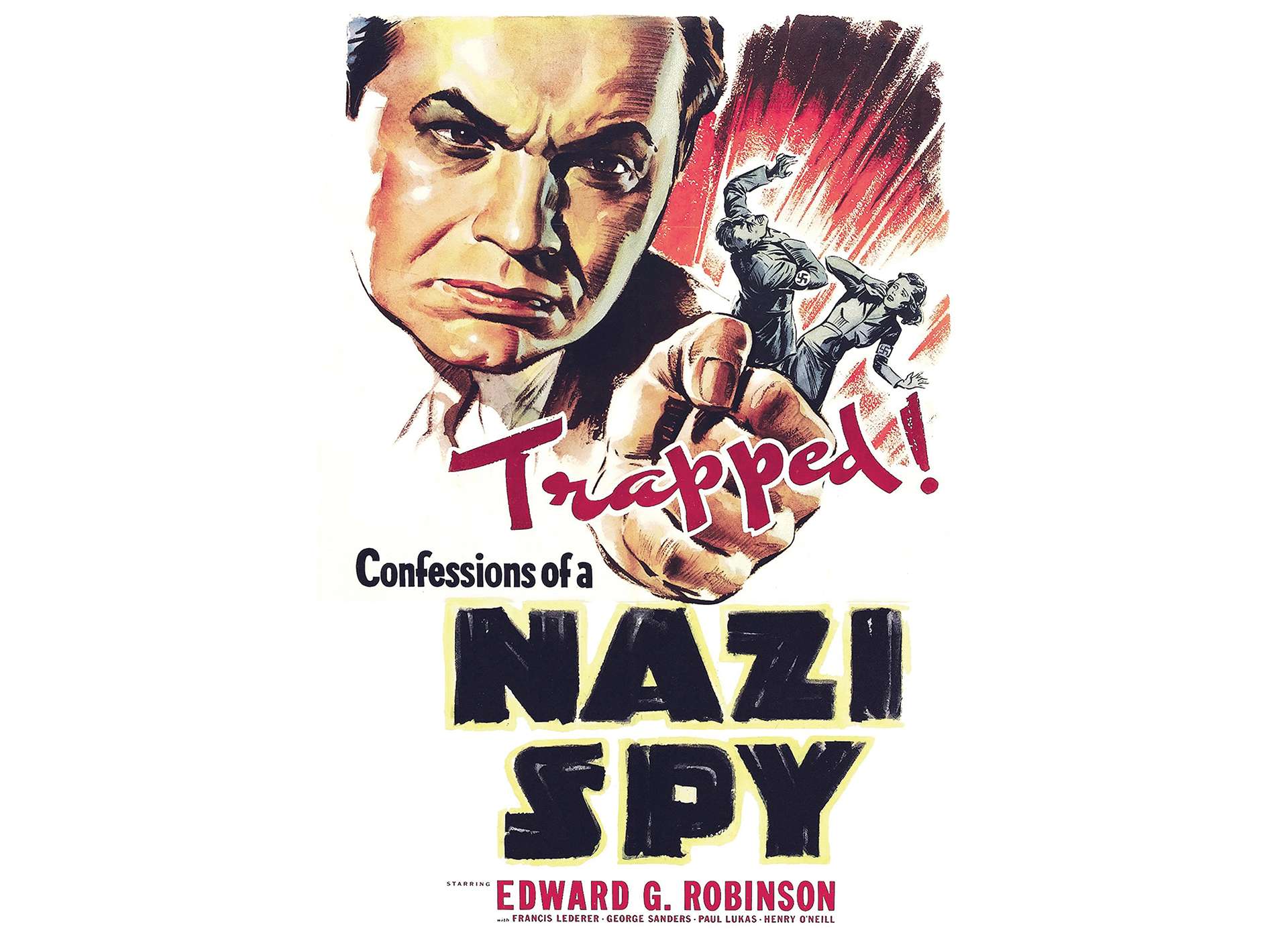This image is an old movie poster for "Confessions of a Nazi Spy" starring Edward G. Robinson. The poster features a dramatic illustration on a white background. Dominating the top half is a menacing man with thick black eyebrows, balding with dark hair on the sides, and wearing a brown suit with a white collared shirt. His clenched fist is prominently thrust forward, creating a sense of urgency and confrontation. To his right, a scene unfolds with a graphic depiction of a terrified woman and a man who appears to be recoiling in shock, wearing a gray Nazi uniform with a swastika armband.

A vibrant red curtain frames the background, creating a stark contrast with the grayscale figures. The word "Trapped" is emblazoned in red cursive across the center of the poster, just above the film’s title, "Confessions of a Nazi Spy," which is in bold black letters, outlined in yellow. Below this, the star-studded cast is listed in red text: Edward G. Robinson, Francis Lederer, George Sanders, Paul Lukas, and Henry O'Neill. The poster's gripping visual elements and bold typography effectively convey the intense and suspenseful nature of the film.